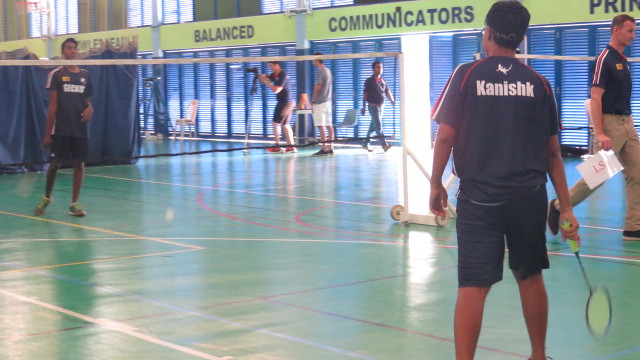In the indoor setting of a gymnasium with green floors, a detailed picture captures an intense badminton game. The focal point features two men in action on the badminton court, each wielding rackets with long handles and neon green netting. Both players are clad in matching blue shorts and short-sleeved shirts adorned with red and white stripes, while one of the shirts bears the name "Kanishk" in white text. In the background, a tall gentleman donning a similar uniform walks past the court, further emphasizing the uniformity and team spirit. Adding to the ambiance, six individuals are visible on the sidelines; some are possibly setting up a camera, and off in the distance, a banner displays the words "Balanced Communicators". The overall scene suggests a well-organized indoor badminton event aimed at promoting the sport.